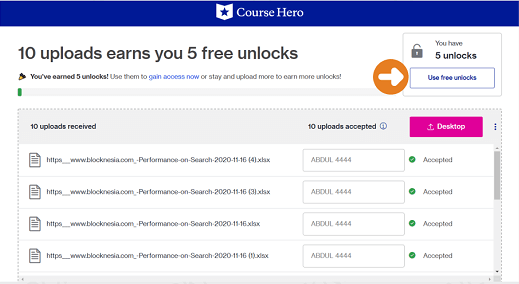The image displays a user interface from Course Hero at the very top, featuring the Course Hero logo which depicts an open book with a star in its center. This logo is set against a blue stripe that spans the width of the screen. Just below this stripe, there is a message stating, "10 uploads earn you 5 free unlocks. You've earned 5 unlocks. Use them to gain access now or upload more to earn more unlocks."

An orange circle with a white arrow inside points towards the option to use the free unlocks, accompanied by text indicating, "You have 5 unlocks." To the right of this, there is an icon of a padlock. Below this section, the interface displays a list of uploaded files with statuses. It shows entries like "10 uploads received" and "10 uploads accepted," and allows the user to click on "desktop" to presumably select or view more files. 

A detailed list of uploaded files is visible, showing their acceptance status. The four files visible on the screen are all marked as "accepted," each denoted by text and a green circle with a white checkmark inside, symbolizing successful acceptance. This interface section clarifies that the user is uploading and managing files, with a clear visual indication of their status.